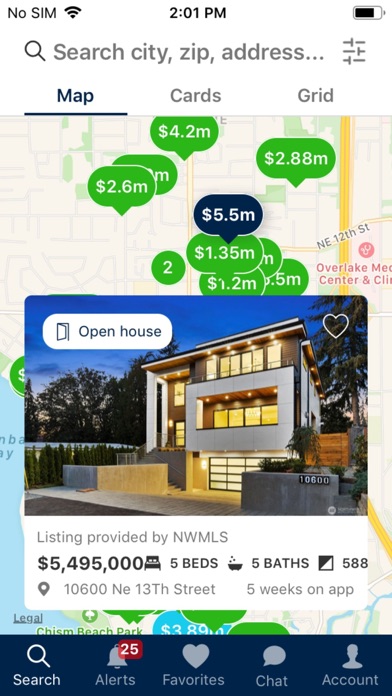A screenshot from a real estate app on a mobile device is displayed. The top of the screen shows standard mobile interface elements: black text on the top left indicating connectivity, the cellular signal icon, the current time of 2:01 p.m. in the center, and the battery life indicator on the top right. Below these, a search bar is prominently positioned, featuring a magnifying glass icon on the left with the placeholder text "Search City, Zip, Address" in gray. On the right side of the search bar is an icon for filter options.

Beneath the search bar, there are three selectable tabs: "Map" (currently selected), "Cards," and "Grid." A map occupies the main section of the screen. In the bottom left corner of the map, a body of water is visible. The map displays several streets, including North East 12th Street towards the top running horizontally. The map also features green bubbles indicating property prices, except for one highlighted bubble in black or dark blue, which displays a price of $5.5M. 

A pop-up overlay partially obscures the map, providing detailed information about the selected property. This includes a photo of the property, the message "Listing provided by NWMLS," and a listed price of $5,495,000. The property details read as follows: five bedrooms, five bathrooms, and 588 (possibly square feet). The address is listed as 10600 Northeast 13th Street, with a note stating the property has been on the app for five weeks.